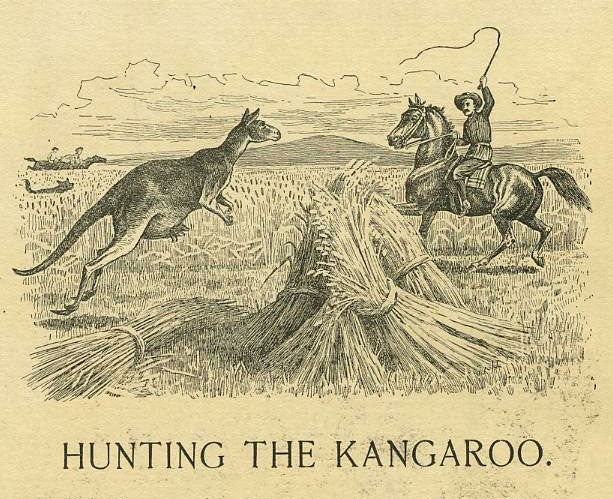In this vertical, sepia-toned sketch rendered in black ink or pencil on coarse-grained beige paper, a dynamic colonial Australian scene unfolds. Dominating the left side of the foreground, a kangaroo on its hind legs, possibly leaping or leaning to the right, displays a long tail extending downwards and two small front paws. This kangaroo has a visible pouch that may even contain a baby joey. Facing the kangaroo from the right, a man in his thirties with a mustache and a round-brimmed hat rides a dark-colored horse. The man’s left arm is raised, holding a long whip, poised as if about to crack it. His horse, depicted with a black mane and tail, trots mildly across the field. The saddle is covered with a plaid blanket.

In the background, amidst a field of stalks resembling barley or wheat, additional details emerge. Two black horses ridden by two Caucasian men and a dark-colored dog are partially visible on the left side. Gray hills and horizontally lined clouds stretch across the horizon. The foreground features loosely heaped bound stalks of grain forming a near-pyramid shape, creating a contextual frame for the scene. Below this meticulously crafted image, the caption "HUNTING THE KANGAROO" appears in capitalized black letters, possibly in Times New Roman font, anchoring the visual narrative.